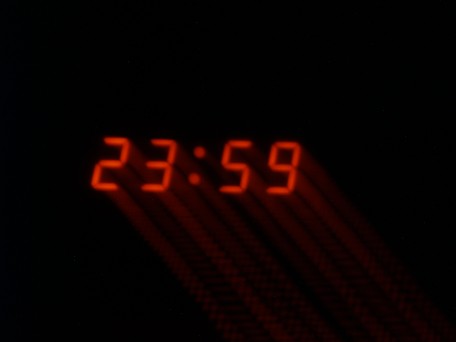The image showcases the face of a digital clock, displaying the time "23:59." The clock appears to have been recently moved, as indicated by red lines underneath the numbers, suggesting motion. The time format hints at a 24-hour system, typically used in digital clocks or timers. The numbers are relatively small, and the red lines to the left and right beneath the digits accentuate the sense of recent movement.